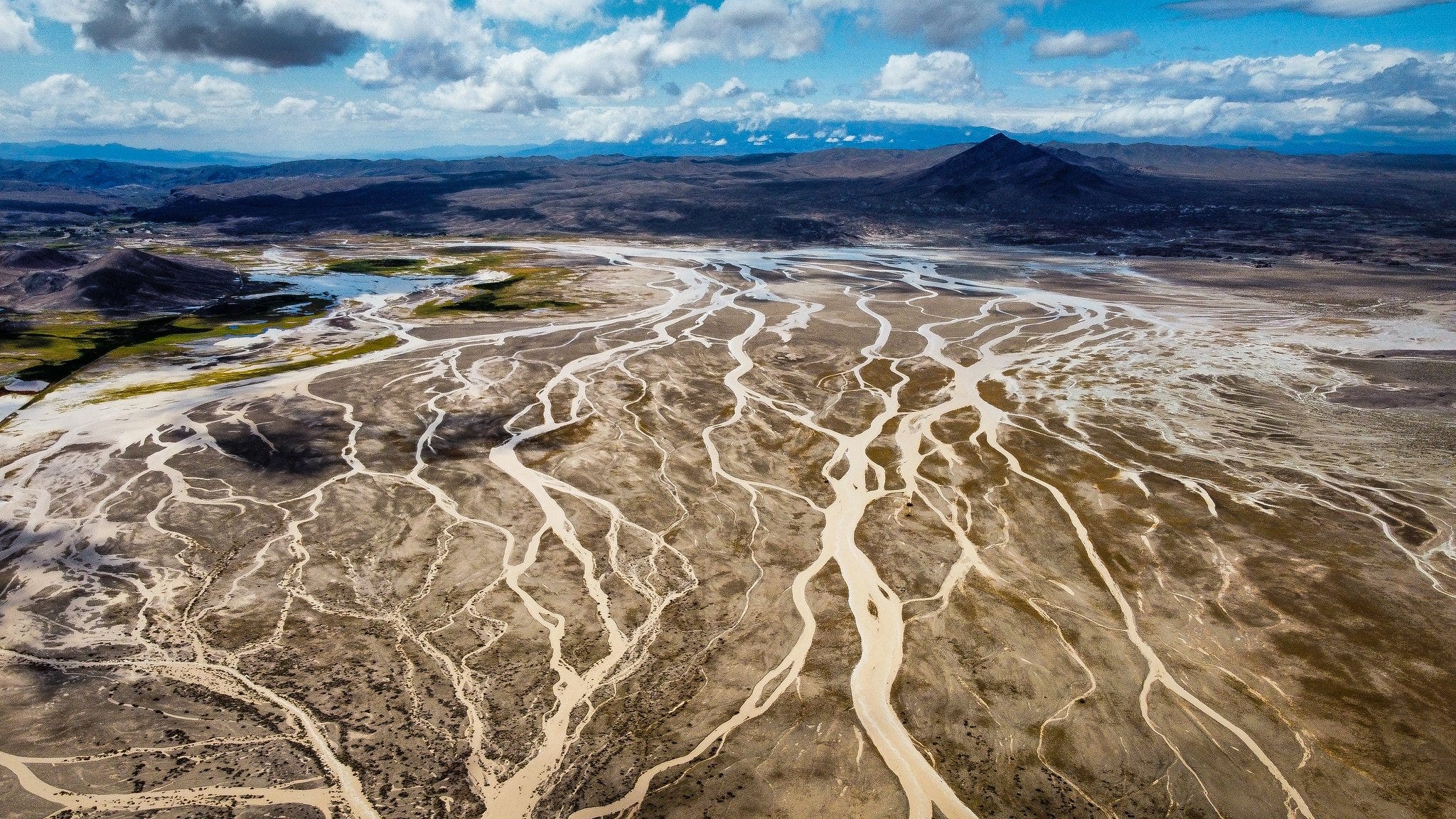This aerial photograph captures a vast, desert-like landscape with a complex network of dried-up riverbeds or eroded waterways stretching across the ground, resembling veins or lightning bolts. The terrain is predominantly brown or tan, with the waterways appearing lighter than the surrounding earth. In the distance, a mountain range looms under a sky that transitions from light blue at the horizon to a deeper blue higher up, dotted with white and gray fluffy clouds. Toward the left side of the image, there's a smaller body of water accompanied by patches of yellowish-green vegetation. The scene is illuminated by sunlight, especially evident in the foreground, while shadows from the clouds add depth and contrast to the mountainous areas in the background.